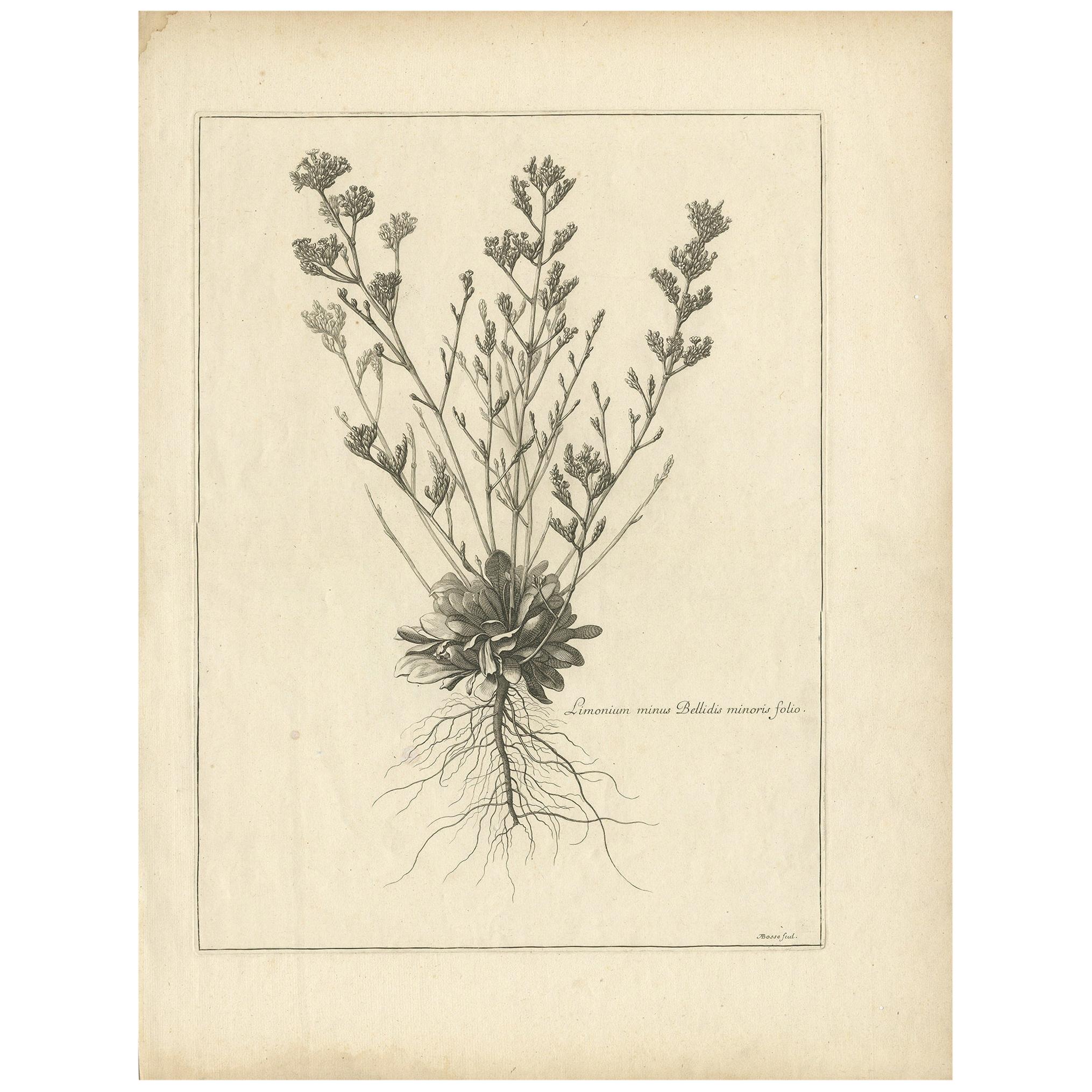The image depicts a vintage yellowed page from a Victorian-era natural history book, featuring an intricately detailed, black and white hand-drawn illustration of a plant species. The rectangular page, oriented vertically, is encapsulated within a light-black, rectangular border. The artwork showcases a plant with a detailed root system at the bottom, consisting of a long main root with numerous thin, squiggly lateral roots extending from it. Above the root, there is a cluster of green leaves, seamlessly leading into long stalks. These stalks exhibit various small buds and seed-like structures, reminiscent of baby's breath. To the left of the plant, there is a cursive label, likely displaying the Latin name of the plant, beginning with "Limonium bellidas minus minoris folio." The overall composition highlights the delicate and precise botanical artistry typical of the period.